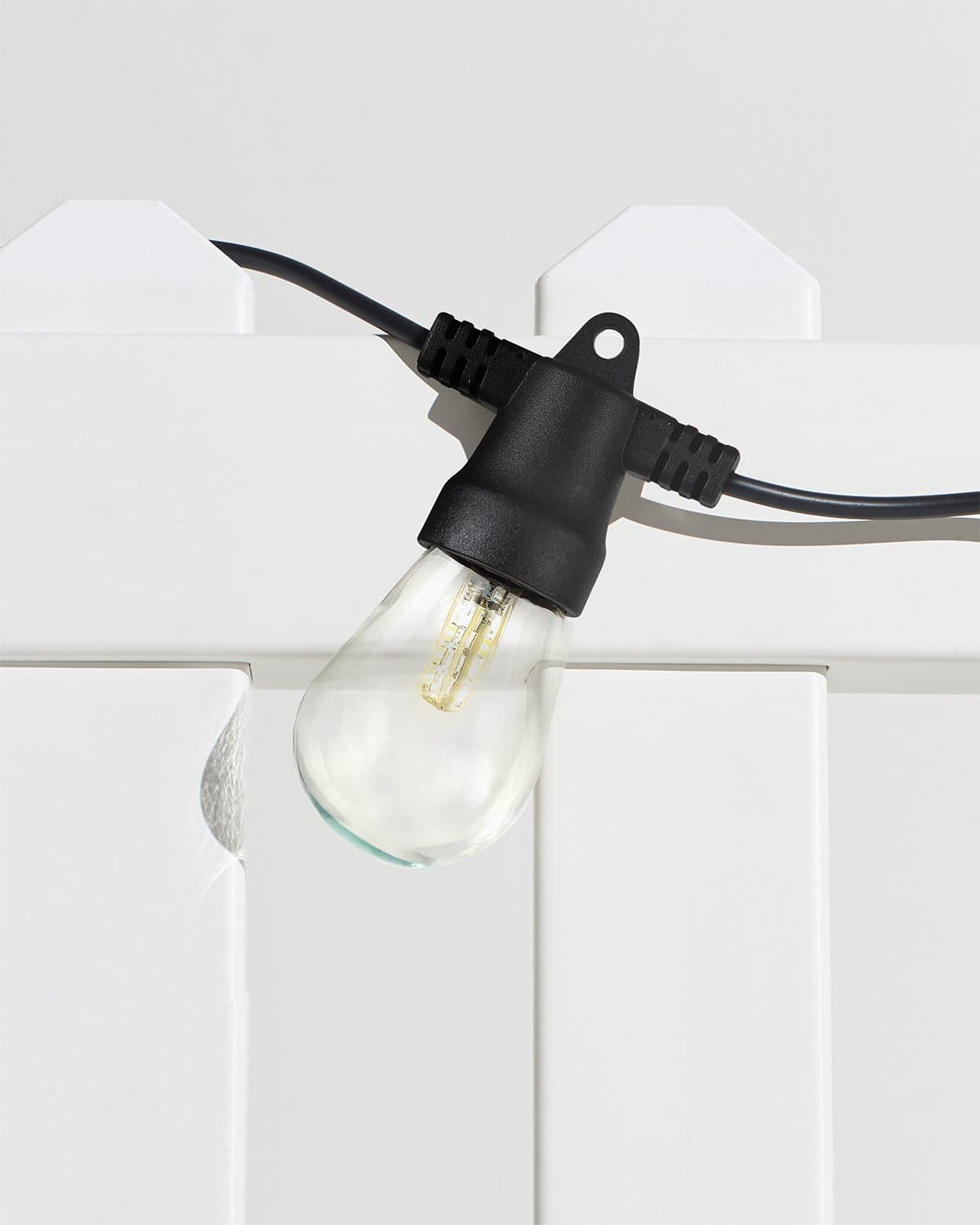The image depicts a non-traditional lightbulb with a smoother, less curved shape at the base, plugged into a black socket. The lightbulb contains a clear glass with a golden filament inside. The socket is connected to black cords extending from both ends. The entire setup is draped over what appears to be a white fence or railing, which has two vertical posts and a horizontal bar at the center, resembling a small gate or crib railing. The background is light gray, possibly a wall, and shadows from both the lightbulb and the cords cast onto the white fence, adding depth to the scene.